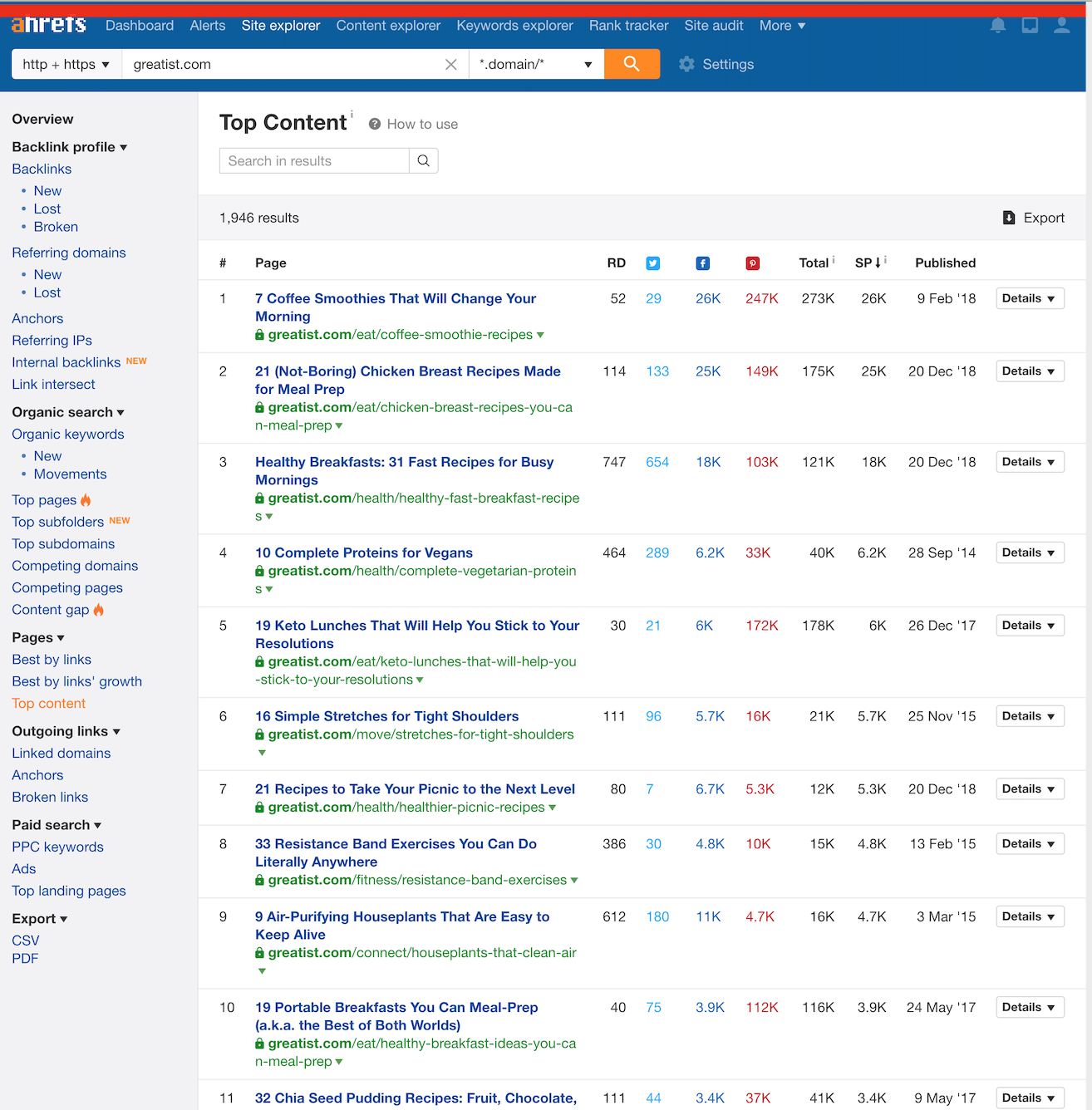The image displays a screenshot of the Ahrefs website interface. At the top, there's a prominent red band that covers part of the Ahrefs logo, making it difficult to discern whether the character underneath is an "H" or an "N." A thicker blue band lies beneath, containing several menu options: Dashboard, Alerts, Site Explorer, Content Explorer, Keyword Explorer, Rank Tracker, Site Audit, and a "More" dropdown menu. To the right of these menus are icons for notifications, a square (likely for multi-functional use), and a person (user profile).

Adjacent to these icons, there's a search bar with a dropdown option for HTTP and HTTPS selection. To the right of the search bar, another dropdown menu allows users to specify the domain type, coupled with an orange button housing a magnifying glass icon, indicative of the search function. The Settings option is located next to this search area.

On the left sidebar, a comprehensive menu lists various functions, beginning with Overview, Backlink Profile, followed by sub-options such as Backlinks, New, Lost, Broken, Referred Domains, New, Lost, Anchors, Referring IPs, and Internal Backlinks. Further options include New List and Intersect.

In the main content area, there’s information about page results, displaying multiple outcomes with titles such as "7 Coffee Smoothies That Will Change Your Morning" and "21 Not Boring Chicken Breast Recipes Made for Meal Prep," along with a count of 1946 results.